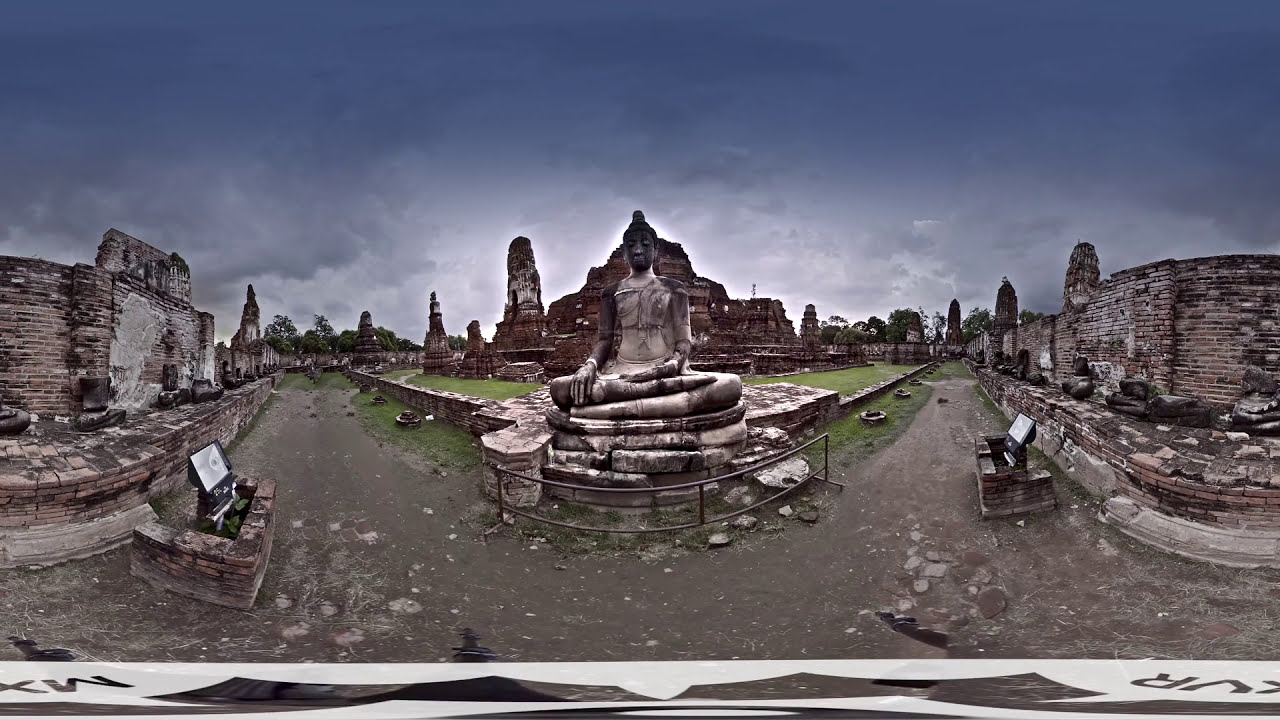The image depicts a serene yet haunting scene of an ancient Buddha statue seated cross-legged in the center of a partially preserved but predominantly deteriorating temple complex. The Buddha statue, crafted from aged stone and adorned with a distinct pointy hairdo, exudes an aura of timeless peace and tranquility. The surrounding area is a panoramic view of the temple grounds, where the dirt path meanders, possibly curving due to the panoramic effect of the photo.

Flanking the statue are substantial stone walls, their surfaces weathered and crumbling, reminiscent of the grandeur of the Roman Colosseum. These decrepit structures suggest a once-majestic edifice now reduced to evocative ruins. Signs on either side of the statue, mounted on bricks, provide visitors with historical context and details about the site. 

The backdrop features a lush green grass patch that transitions into more dilapidated ruins, hinting at a once flourishing temple complex. The reddish hue of the ruins contrasts with the somber, gray-tinged sky that looms overhead, suggesting an impending storm. Hidden amid the ruins is a towering structure that could be the remnants of a significant building, possibly a place of worship such as a cathedral or a temple, standing as a silent testament to the past. Overall, the image captures the fascinating juxtaposition of serene religious artistry set against the raw, untamed beauty of a decaying historical landmark.